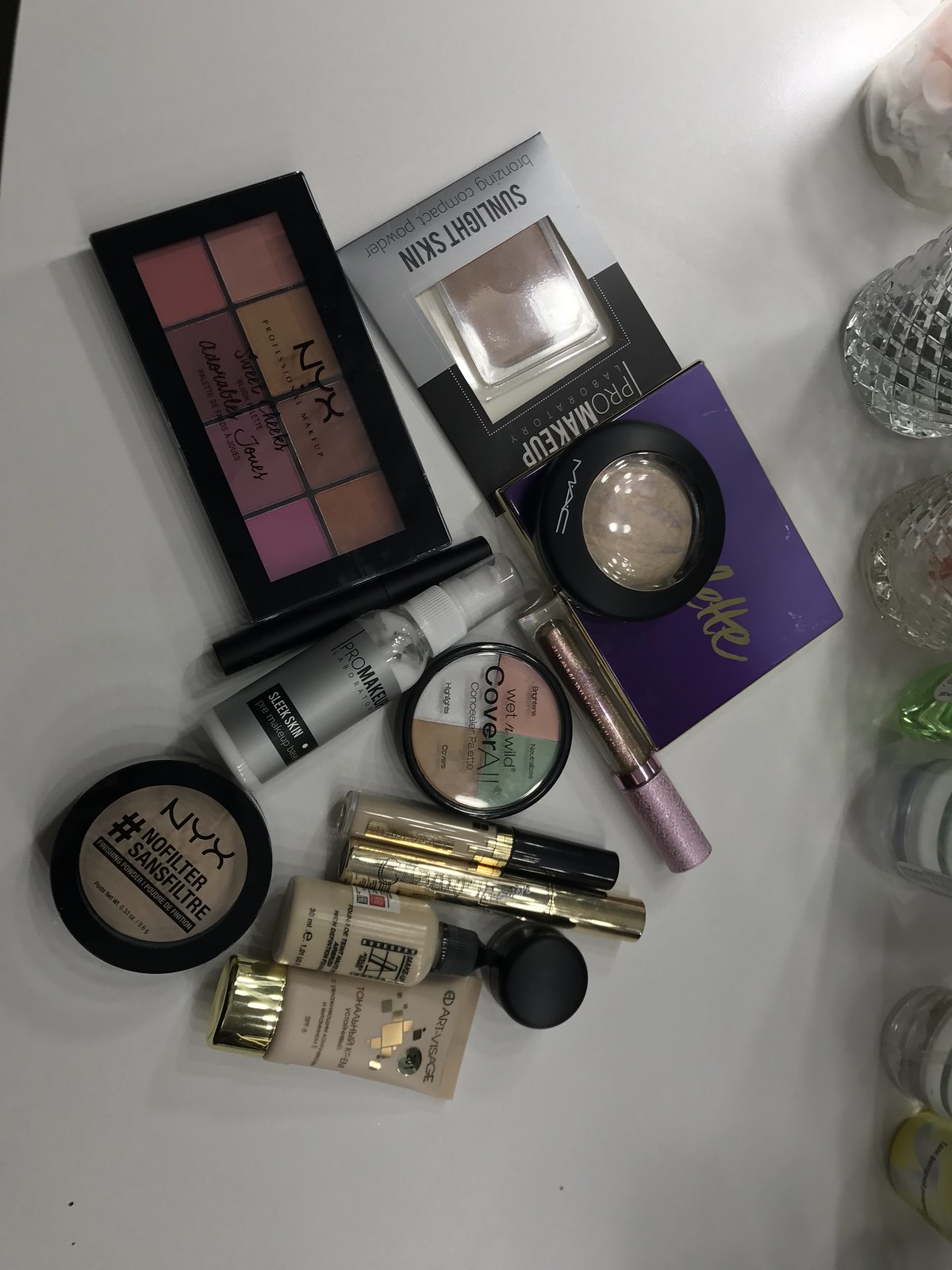This photograph features an assortment of makeup items meticulously arranged on a countertop, albeit rotated 90 degrees to the right. Along what is now the right-hand side of the image, we observe several clear glass candle holders, some adorned with a diamond-shaped pattern. There are approximately five or six of these candle holders, likely intended for small tea light candles.

In the upper left corner of the image, there is an NYX Professional Makeup eyeshadow palette with eight shades, predominantly in pink and plum hues, labeled "Sweet Cheeks, Adorable Tones." Adjacent to this palette is an upside-down Pro Makeup Laboratory compact, labeled "Sunlit Skin Bronzing Compact Powder."

Positioned below the bronzing powder is a blue MAC palette. The palette itself is encased in a blue cardboard, with the actual container being black and containing a white powder. Scattered around the central area of the photograph are several lip gloss tubes, one distinctly purple, with the others in traditional lip gloss forms whose exact shades are indeterminate.

Additionally, there is a small bottle labeled "Pro Makeup Laboratory Sleek Skin," the specifics of which are not entirely clear. Nearby is a Wet n Wild Concealer palette, characterized by its round shape, black borders, and four distinct colors: peach, green, dark beige, and white. 

At the bottom of the arrangement lies an NYX No Filter Finishing Powder in a round black container, holding a brown-hued product. Completing the collection are two more small bottles of makeup products, one branded "Art Passage." 

Overall, the image is a neatly arranged, diverse display of various makeup products captured on a countertop, showcasing an array of colors and brands.